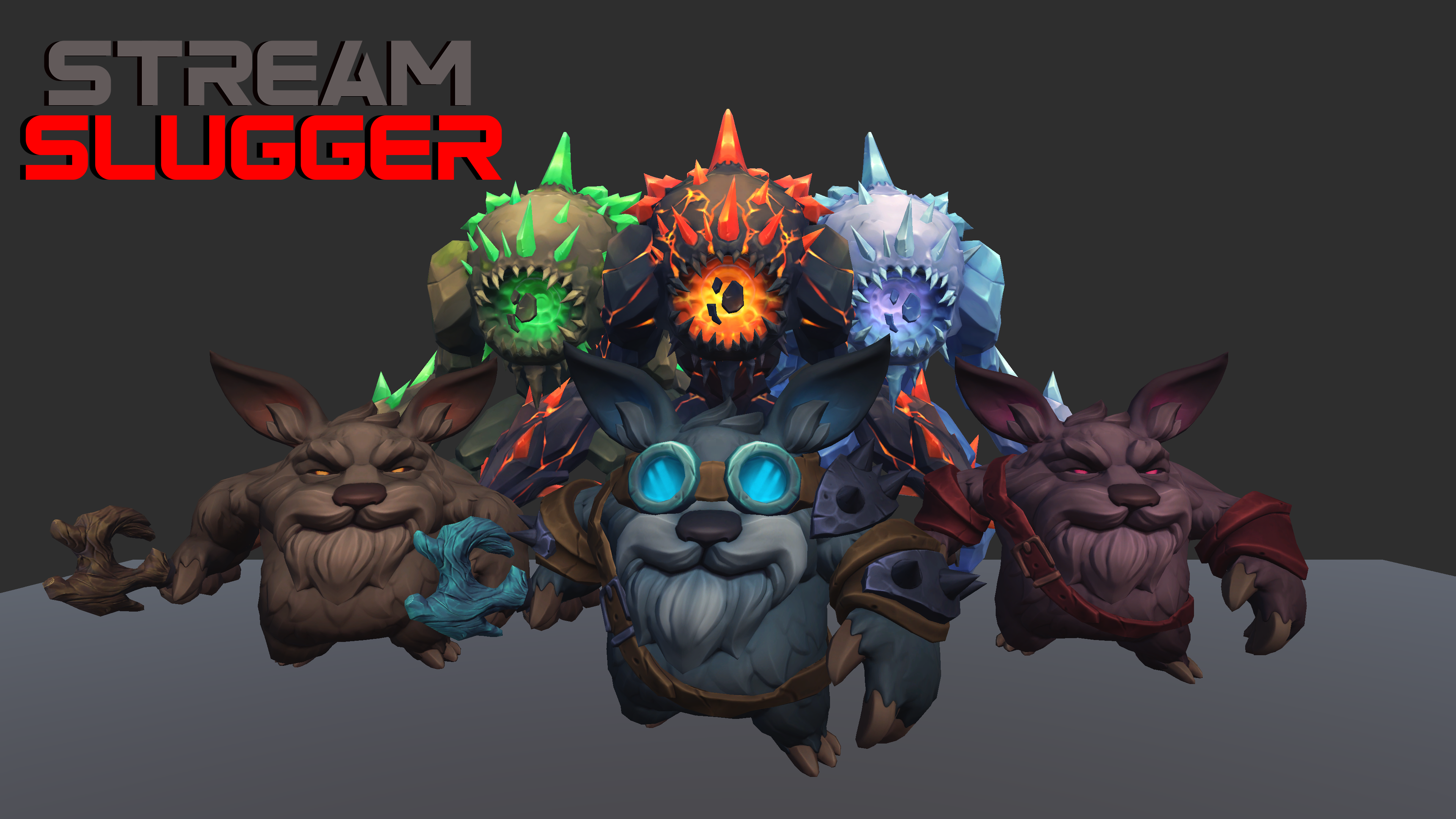In a dark gray background that transitions from darker tones at the top to lighter shades at the bottom, an animated scene unfolds featuring six distinct, 3D, cartoon-like characters. The top left corner bears the text "Stream Slugger," with "Stream" in gray and "Slugger" in red.

The first row comprises three anthropomorphic, furry, dog-like creatures, each standing upright with opposable thumbs. Equipped with axes or wooden clubs, they are clad in leather armor. The center character, dark grayish-blue with blue goggles strapped behind its head, stands flanked by two companions: a burgundy-colored one with glowing red eyes on the right, and a brown-colored one on the left. All three boast large bat-like ears, bearded faces, and stout, fur-covered bodies, complete with three-toed feet and three or four-fingered hands.

Behind them, three towering, one-eyed monstrosities loom. Each sports a distinct color and texture: the leftmost creature is green, the middle one is black with protruding lava-red spikes, and the rightmost is adorned with ice crystals, tinged a purplish-blue. Their grotesque heads resemble gigantic singular eyes, giving them a menacing, otherworldly appearance.